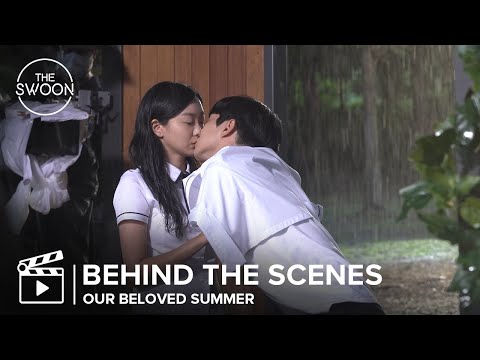In this image, we see a frame from what appears to be a Korean movie or drama titled "Our Beloved Summer." The top left corner of the image features a white circle with the text "The Swoon" inside. At the bottom, just above a black band, there's a movie clipboard icon with the text "Behind the Scenes, Our Beloved Summer." The main scene captures a romantic moment between two young, Asian individuals with black hair and olive skin. The girl, who has long black hair and is wearing a white short-sleeve shirt, is seated. The boy, with short black hair and a white long-sleeve shirt, leans in to kiss her. Her hand is gently placed on his chest or arm, though it is partially obscured by his shirt. They are inside, suggested by some wooden panels and furniture on the left, but through a window in the background, you can see it's raining outside, revealing trees and green grass.